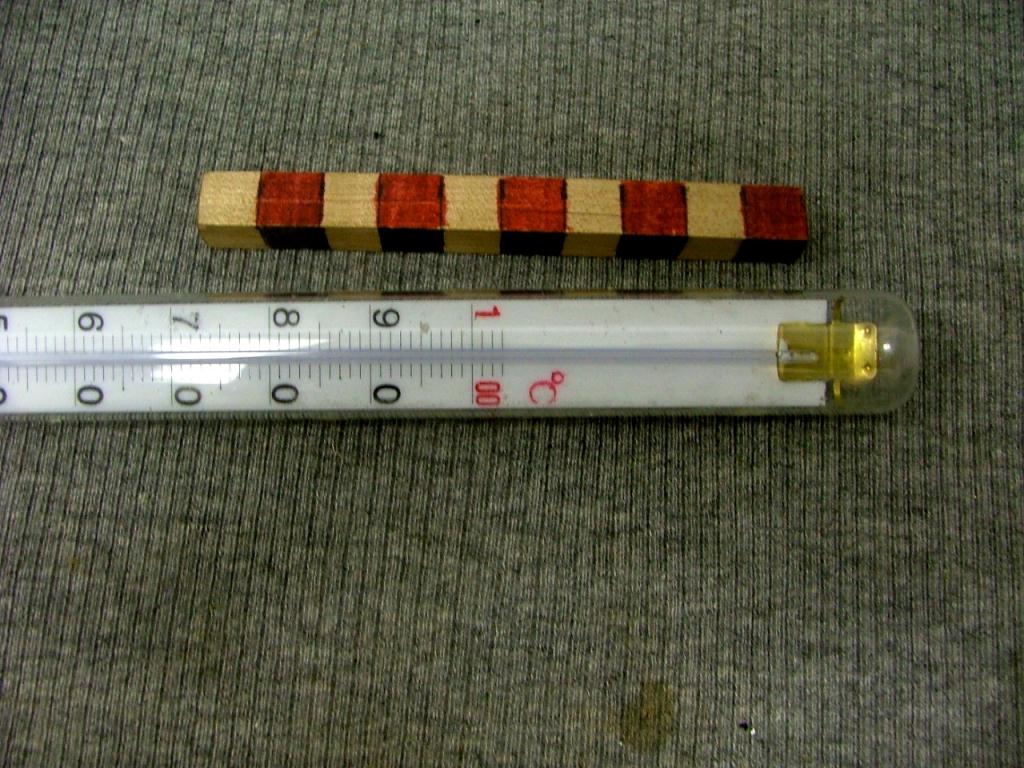The photo features a horizontally placed wooden stick that is decorated with thick stripes of alternating colors: starting from the right tip, red and tan repeat in sequence until the unpainted section at the left tip. The stick, square-shaped at the top, rests on a ribbed gray fabric. Directly below the stick lies a prominently large, round thermometer resembling a candy thermometer, characterized by its very wide and clear circular face. The thermometer has a gold screw holding it in place inside its glass tube. The top of the thermometer is positioned towards the right, with the numerical markings running horizontally and appearing backward from the top to the middle. Also noticeable is a small, round brown stain located towards the bottom right of the image, suggesting a spill or spot on the fabric.